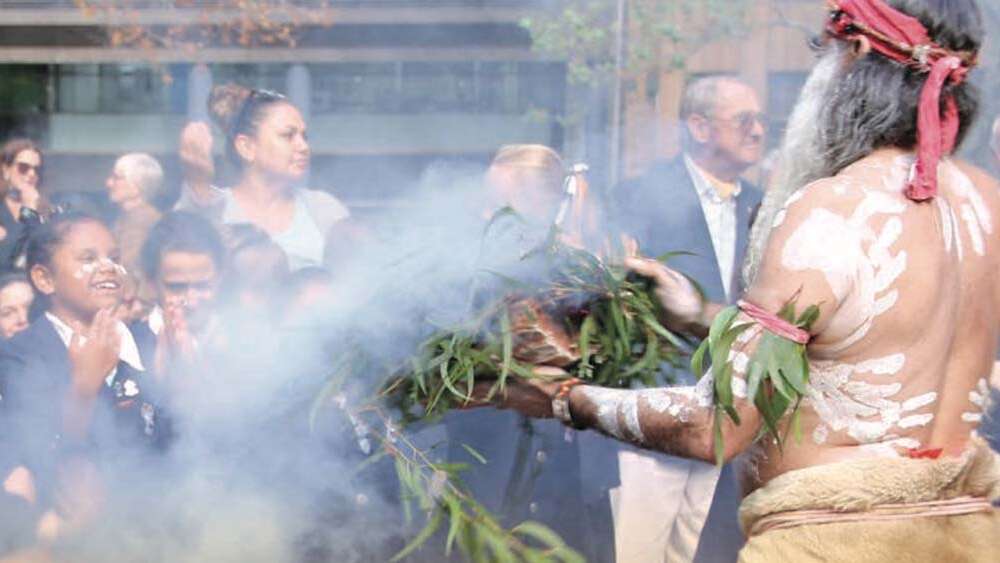In this detailed image of a vibrant tribal ceremony, a shirtless, elderly man with a long white beard and gray hair takes center stage. Adorned in an animal hide skirt secured by a pinkish rope around his waist, he also sports a red piece of rag tied around his head and another piece of red rope around his upper arm, which holds green leaves beneath it. His body, back, and arms are covered in white painted handprints, enhancing his ritualistic appearance. The man holds a large bundle of green leaves in his left hand, emitting visible smoke. Surrounding him is a diverse crowd of children, adults, and elders, all with slightly darker skin tones. Among them, notably, a girl with white face paint smiles with her mouth open. The background features a structure that covers the entire area, providing a backdrop to the ceremonial scene.